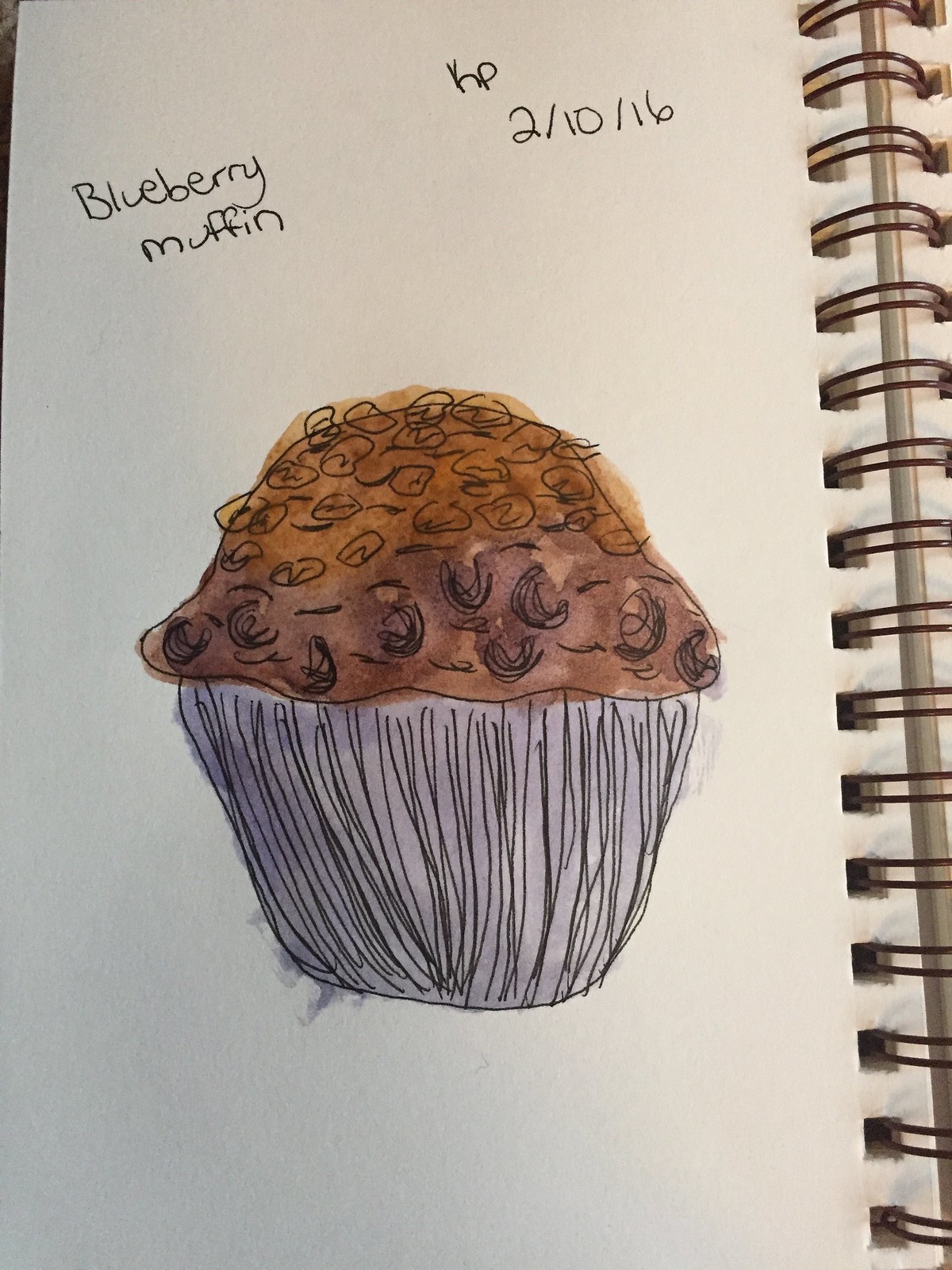This photograph captures a page from a ring-bound sketchbook, highlighting a detailed pen drawing labeled "Blueberry Muffin" at the top right, in handwritten pen. The drawing is dated and signed "KP 2-10-16." The sketch features a visually appealing depiction of a blueberry muffin, characterized by its intricate pen striations that illustrate the muffin's paper wrapping. The muffin top is artistically rendered in brown watercolor, while the wrapper is painted in varied shades of gray watercolor. The drawing prominently displays a blobby shape with sketched details suggesting raisins or blueberries, showcasing the artist's detailed and textured approach. The ring bindings of the sketchbook are visible on the right side of the image, providing context and framing the artwork within the page.